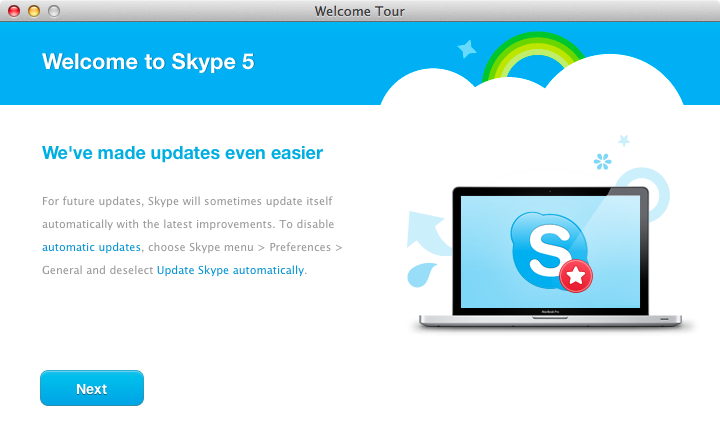In this promotional image for Skype 5, a welcoming message prominently features the text "Welcome to Skype 5. We've made updates even easier." The message explains that future updates will occasionally be installed automatically to provide users with the latest improvements, while offering instructions on how to disable this feature by navigating to the Skype menu, selecting Preferences, choosing General, and then deselecting "Update Skype Automatically."

The visual aesthetics of the image include a harmonious palette of blue and white. To the right side of the image, a MacBook is displayed, showcasing the Skype logo accompanied by a white star set against a red circle. The overall color scheme further extends into shades of green, red, yellow, and variances of blue and white, bringing a vibrant and engaging visual experience to the viewer.